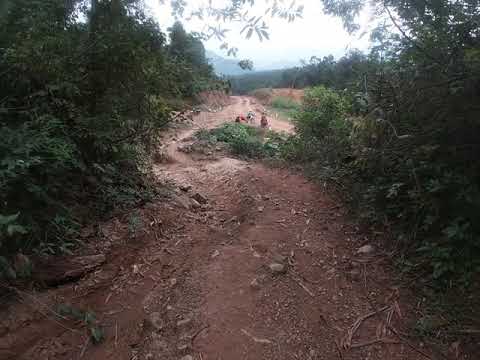The photograph captures a narrow, rough dirt path with a light red, clay-like hue, winding through a densely foliated area. The scene is bright, though the sun isn't directly visible, giving the atmosphere a diffuse light. A rich, lush green canopy from bushes and low trees tightly flanks both sides of the path, with some leaves encroaching into the upper frame of the image. The path is strewn with small rocks, sticks, and twigs, adding texture to its surface. In the distance, the path curves gently to the left and is partially obstructed by a continuation of thick green shrubbery. Farther ahead, three indistinct figures, possibly people, stand where the path meets a broader dirt road. This junction is framed by earthen embankments and more foliage, which also appears to rise into a slight hill, giving a subtle hint of elevation in the background.